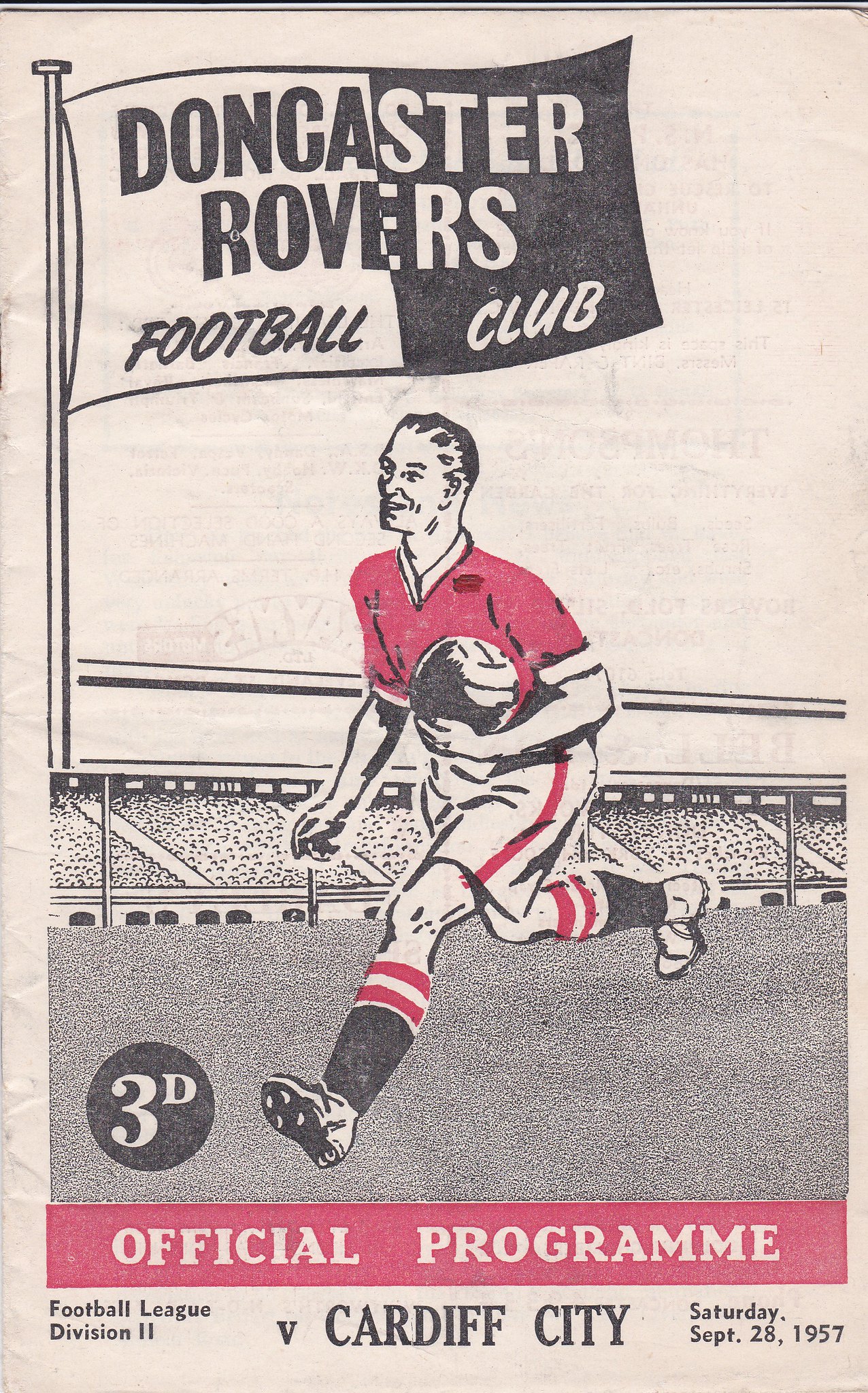The front page of this game day program for Doncaster Rovers Football Club, dated Saturday, September 28, 1957, is a striking composition of black, white, and red. Dominating the top of the cover, a flagbearing the club's name is split into a black and white design, with 'Doncaster Rovers Football Club' displayed in contrasting text across the halves. Below this, an illustrated soccer player wearing a red jersey with white trim, white shorts with red stripes, and black socks with red and white accents is depicted in mid-run, holding a soccer ball close to his body. The background reveals a packed stadium, emphasizing the event's significance. At the bottom left corner, a black circle marked '3D' hints at the publication's edition or price. Stretching across the bottom of the cover, a red banner with white text proclaims 'Official Program,' while below this, in smaller black text, the details 'Football League Division II vs. Cardiff City' affirm the match information.